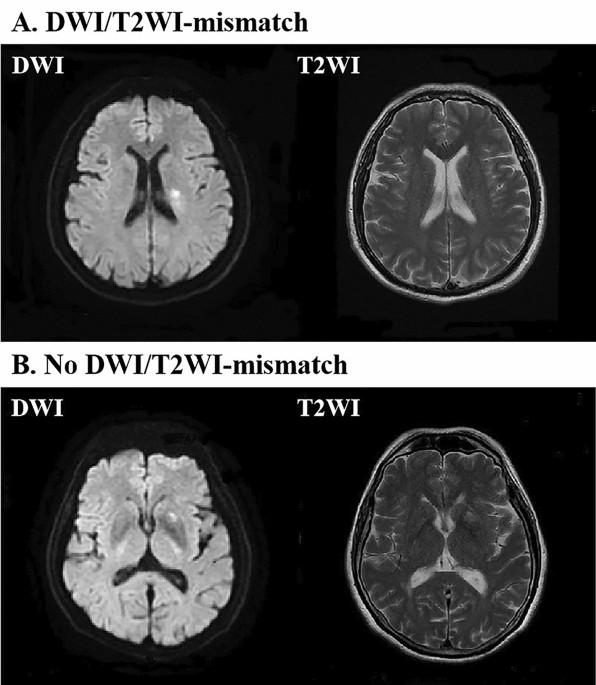This image presents two sets of brain MRI scans labeled A and B, each comprising a pair of images. In set A, which is described as having a "DWI/T2WI mismatch,” the first image (DWI) features a predominantly white depiction of the brain, while the second image (T2WI) contrasts with a darker, grayscale rendering of the same brain structure. Set B, labeled as "no DWI/T2WI mismatch," similarly includes two scans: the first (DWI) is a lighter image of the brain, predominantly white with intricate designs, while the second (T2WI) is darker, with more pronounced black tones and subtle outlines. Both sets are displayed against a black background, typical of MRI scan presentations.